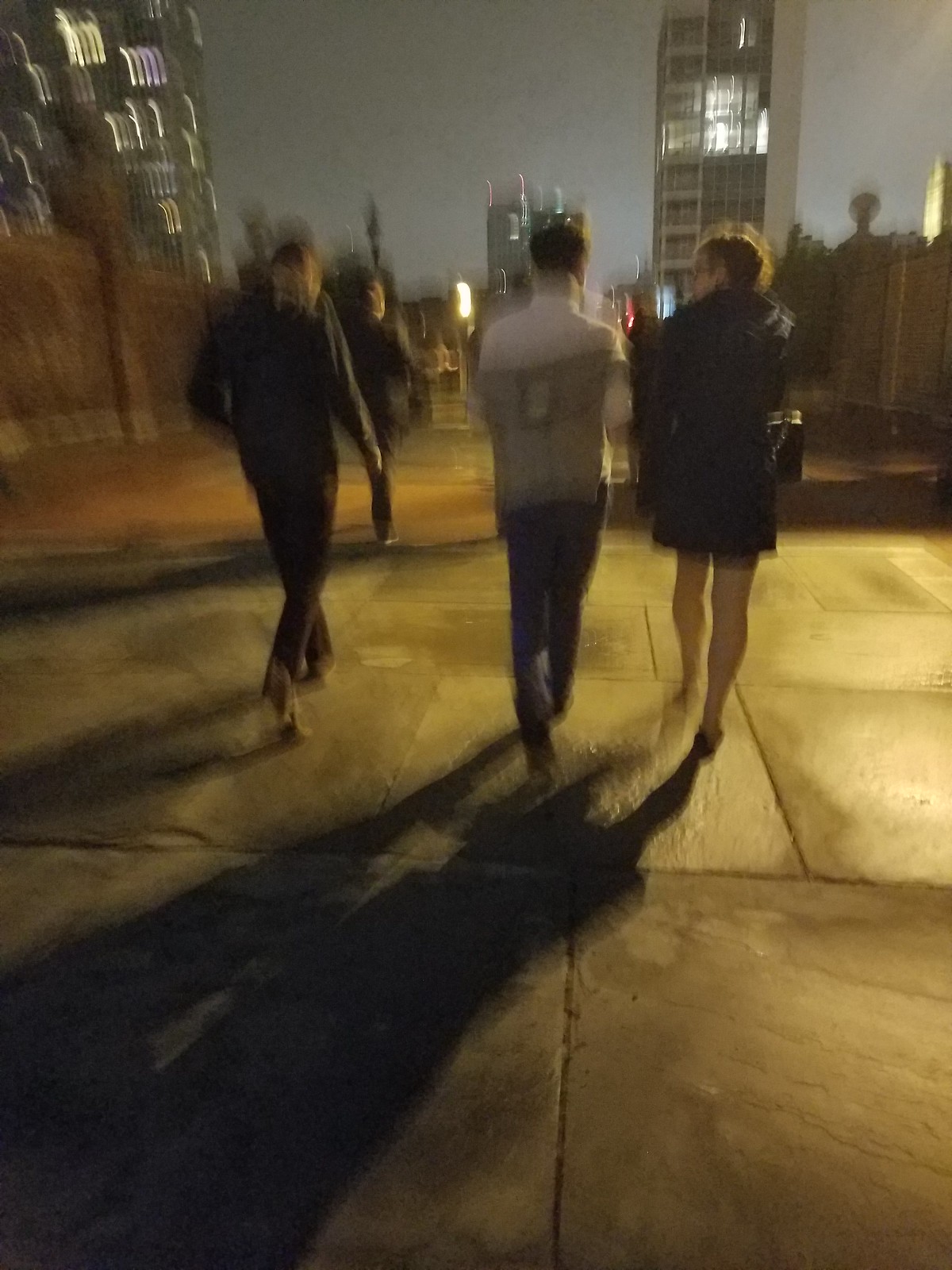The image captures a blurred nighttime scene on a city street or pedestrian walkway made of large gray stone tiles arranged in a two-feet square format. The street is flanked by tall, brownish brick walls, and beyond them, various high-rise buildings can be seen, illuminated with lights in different hues including white, purple, yellow, and green. In the foreground, three people are walking away from the camera. A woman on the left is wearing a warm black jacket, a short skirt, possibly stockings, and carrying a purse. Next to her, a man is dressed in jeans and a white shirt, while another man wearing a black jacket and brown pants is nearby. The scene is lit by streetlights, and the photograph’s blurriness suggests it was taken while the photographer was in motion.